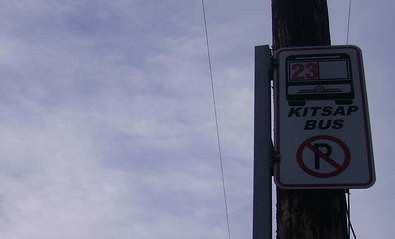A clear daytime sky dominates most of the image, showcasing a light blue hue with loosely scattered white clouds. On the right side of the image, two thin, nearly parallel telephone wires are visible, both of which are black and flank the sides of a large wooden pole. The pole is prominent in the frame, so much so that it’s unclear if the wires actually meet the pole. Attached to the large wooden pole is a smaller metal pole on its left side. This metal pole supports a rectangular sign that is primarily white with black text reading "KITSAP bus" and a black "P," which is overlain by a red circle with a diagonal line, indicating a no parking zone. Additionally, there is an illustration of a bus on the sign, and on the bus window, the number "23" is written in red.